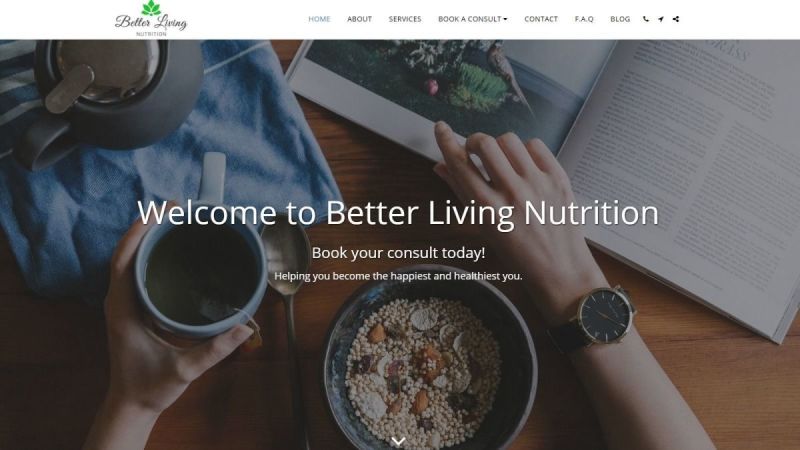This is a screenshot of the landing page for the "Better Living Nutrition" website. At the top left corner, the logo is prominently displayed, featuring the brand name "Better Living" in a cursive handwriting style, accompanied by a green leaf icon symbolizing health and nature. 

The navigation menu spans across the top of the page, offering links to essential sections like Home, About, Services, Book a Consult, Contact, FAQ, and Blog. There are also three small icons to the right of the menu—a telephone, an arrow, and three circles whose function is unclear.

The central feature of the page is a tranquil photograph that spans its width. The image captures a serene breakfast scene viewed from above: a person seated at a wooden table. Their left hand holds a cup of coffee, with a coffee pot stationed nearby, while their right hand flips through a book. Between their hands rests a bowl of muesli, suggesting a healthy and balanced start to the day. 

Superimposed on this calming image is the website's main message. The text "Welcome to Better Living Nutrition" is prominently displayed at the center in large writing. Below it, slightly smaller, is a call-to-action: "Book your consult today." The smallest text, positioned underneath, reads, "Helping you become the happiest and healthiest you." This narrative welcomes visitors and encourages them to engage with the services offered by Better Living Nutrition, aiming to improve their health and happiness.